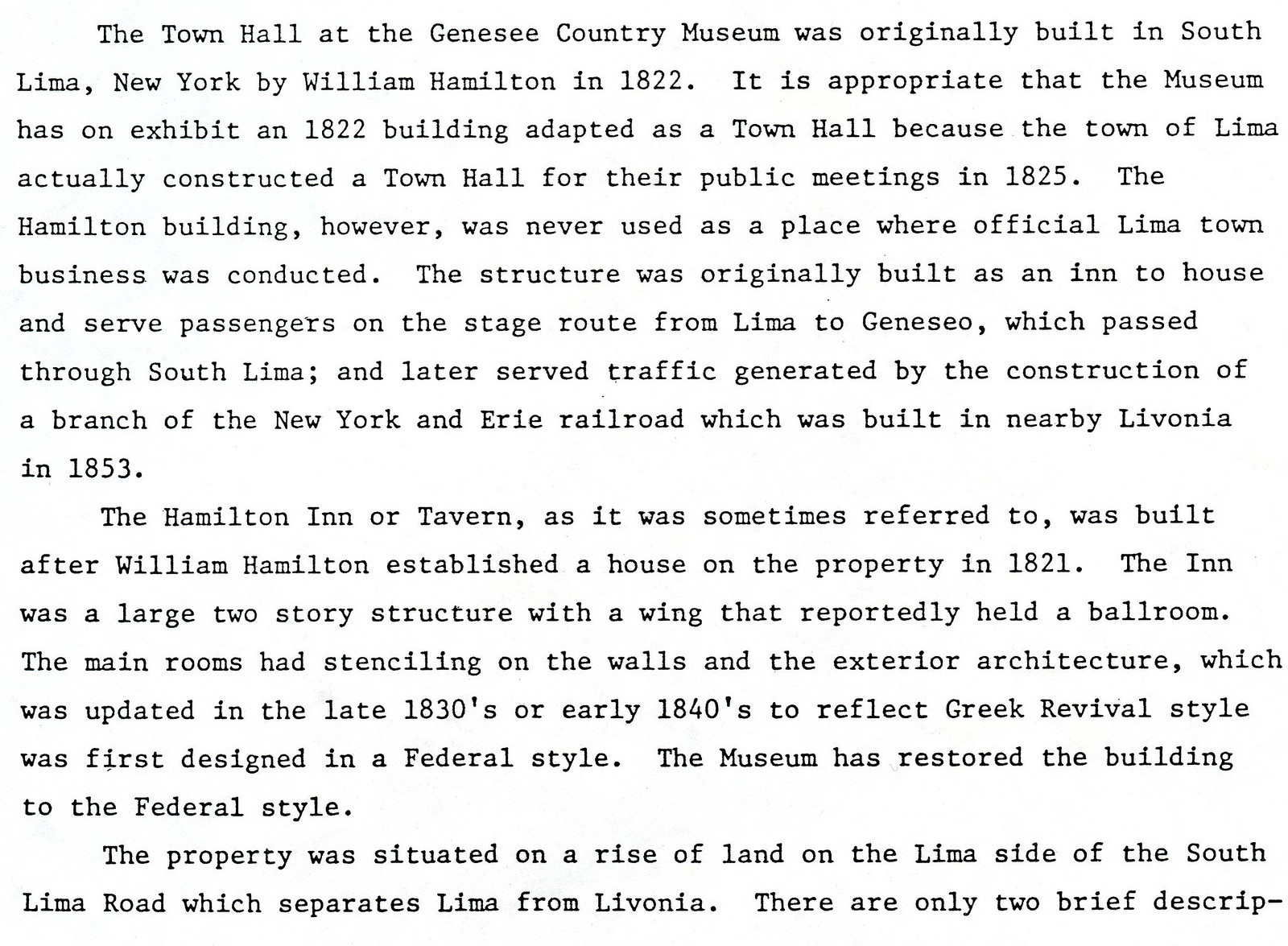This image displays a typed text on a white background, detailing the history of the town hall at the Genesee Country Museum. Originally built by William Hamilton in South Lima, New York, in 1822, this structure has been adapted to serve as an exhibit at the museum. Although the town of Lima constructed their town hall in 1825 for public meetings, Hamilton's building was never used for official town business. Initially constructed as an inn, it served passengers on the stage route from Lima to Geneseo and later traffic from a branch of the New York and Erie Railroad in 1853. Built after Hamilton established a house in 1821, the two-story inn featured a wing that reportedly housed a ballroom, stenciled main rooms, and architecture which transitioned from federal style to Greek revival in the late 1830s or early 1840s. The museum has since restored the building to its original federal style. Located on a rise of land on the Lima side of the South Lima Road, the inn's historical significance is preserved for museum visitors. The text ends abruptly, indicating there may be more to the description.